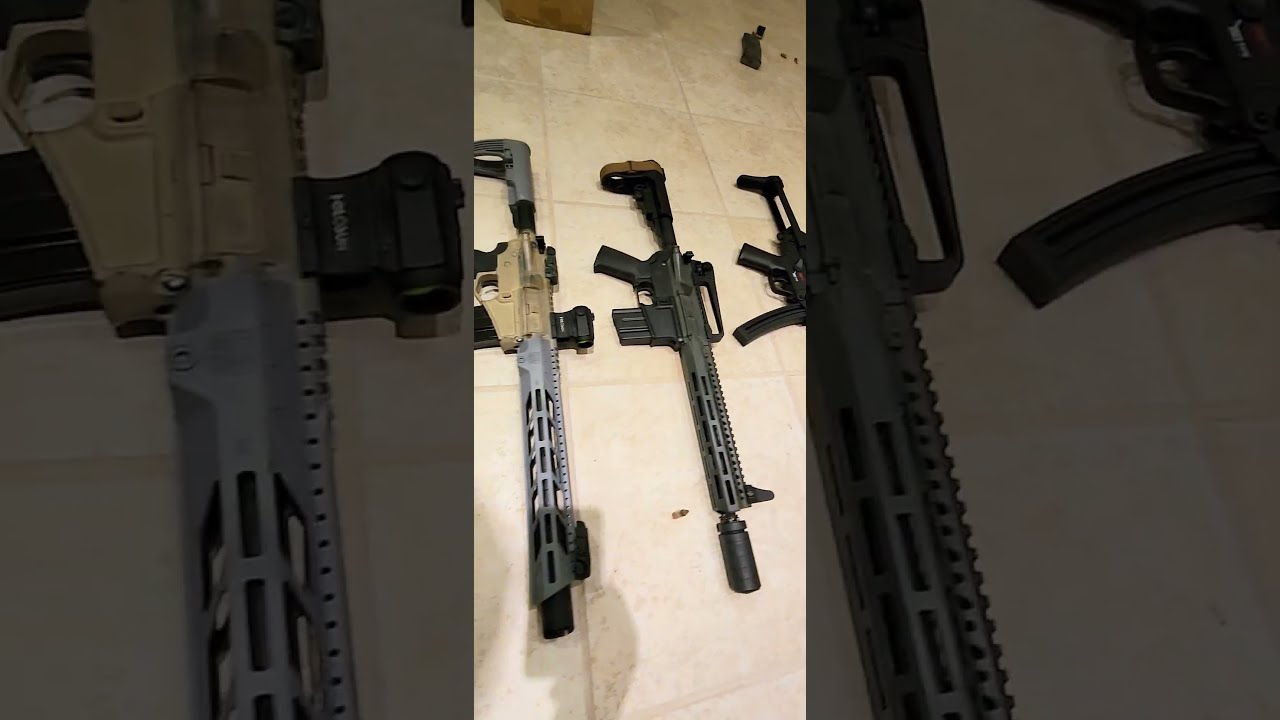The image showcases a collection of three assault rifles arranged on a tile floor. The perspective is from the bullet ends of the guns, emphasizing their lengths and details. The rifle on the left features a silver barrel with a tan handle and trigger area, appearing as the longest. The center rifle is predominantly black with a slight brown accent near the end. The rifle on the right, partially cut off from view, is entirely black. All three rifles have distinct features such as heat guards over the barrels and visible magazines, with the rightmost weapon sporting a curved magazine reminiscent of an AK-47. In the background, there are several scattered bullets, a cardboard box in the upper left corner, and a magazine on the upper right. The image captures the shadow of a person, possibly the photographer, recording with a phone. The setting appears to be either a kitchen or a white-tarp-covered floor, suggesting a casual display, potentially for a gun club or personal collection.